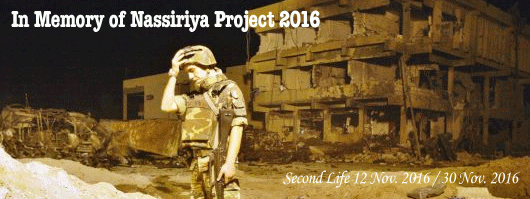In the image, a nighttime scene unfolds with a horizontal layout primarily dominated by a single soldier, slightly off-center to the left. The soldier is depicted from head to mid-thigh, clad in camouflage and looking down somberly with his right hand resting on his helmet, conveying a sense of pain and sadness. His left hand hangs loosely by his side. Behind him lies a three-story building, heavily bombed and partially demolished, exposing its fragmented units and surrounded by scattered rubble. The surrounding area is riddled with debris, implying recent devastation, presumably due to conflict. The image has a sepia tone, adding a yellowish-brown tint that enhances the melancholic and historical feel. In the top left corner, white text reads, "In memory of Nasseria Project 2016," and at the bottom left, it states, "Second Life, 12 November 2016 / 30 November 2016." This poignant scene encapsulates the gravity of destruction and the emotional toll on those who witness it.